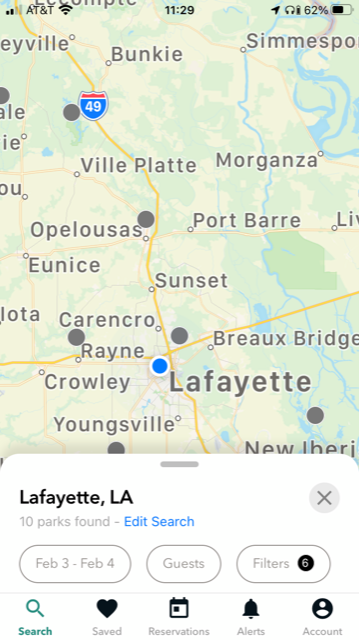Here is the revised and detailed caption based on the provided voice description:

---

This portrait-oriented screenshot showcases a detailed map search highlighting various towns and notable landmarks. Dominating the top half (or more) is a map featuring a diverse landscape marked by towns, waterways, and brown patches of land. Prominent towns visible on the map include Bunky, Ville Platte, Organza, Port Barre, Sunset, Eunice, Currents Crow, Rain, Crowley, Youngsville, and notably Lafayette, which is denoted by a blue dot, suggesting it might be the primary focus. This particular map area seems to be somewhere in Louisiana. The map is interspersed with numerous railroad lines, with two intersecting near the bottom, along with the route number 49.

Beneath the map, there is a draggable, white pop-up box in landscape orientation featuring black and gray text. It prominently displays "Lafayette, LA" in black font, followed by a gray line stating "10 parks found," and a blue link that reads "edit search." The box also contains bubbles to input dates displaying "February 3rd to the 4th," details about "guests," and search "filters." A small black circle with a white number "6" appears within the filter bubble. Below these elements, there are icons for "search," "saved," "reservations," "alerts," and "account," with the "search" icon highlighted in blue.

---